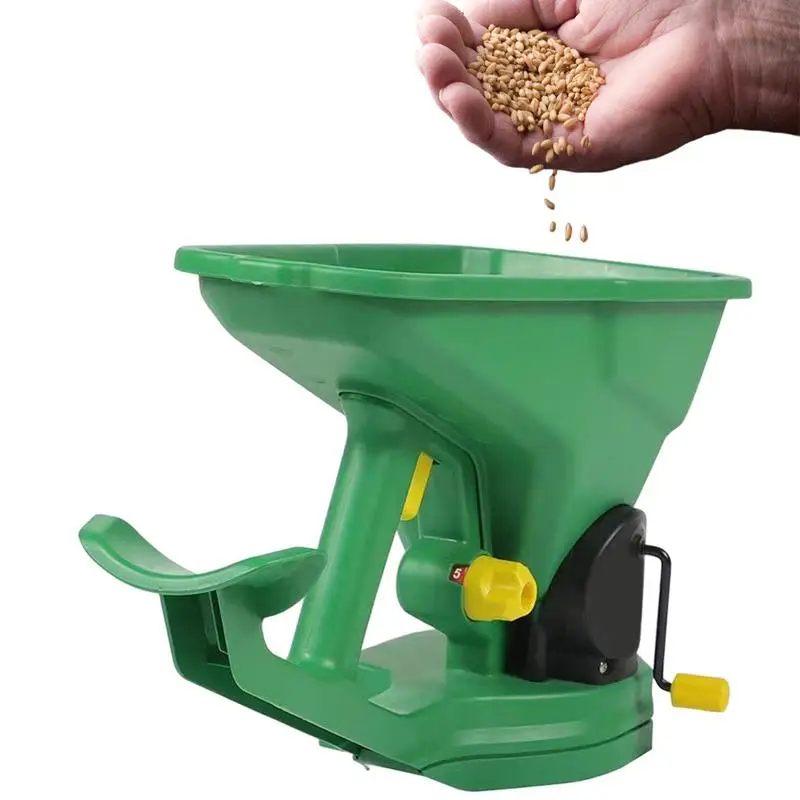The image depicts a small, green plastic grain grinder with a round base and an open top that resembles a bucket. A hand is positioned above the grinder, pouring brown grains, possibly rice or grain kernels, into the square opening at the top. The grinder features a black handle with a yellow knob, designed for manual turning to process the grains. The background is a plain white color, emphasizing the machine's bright green hue. The grinder's compact size suggests it can only produce a limited amount of ground grain, making the process potentially time-consuming.